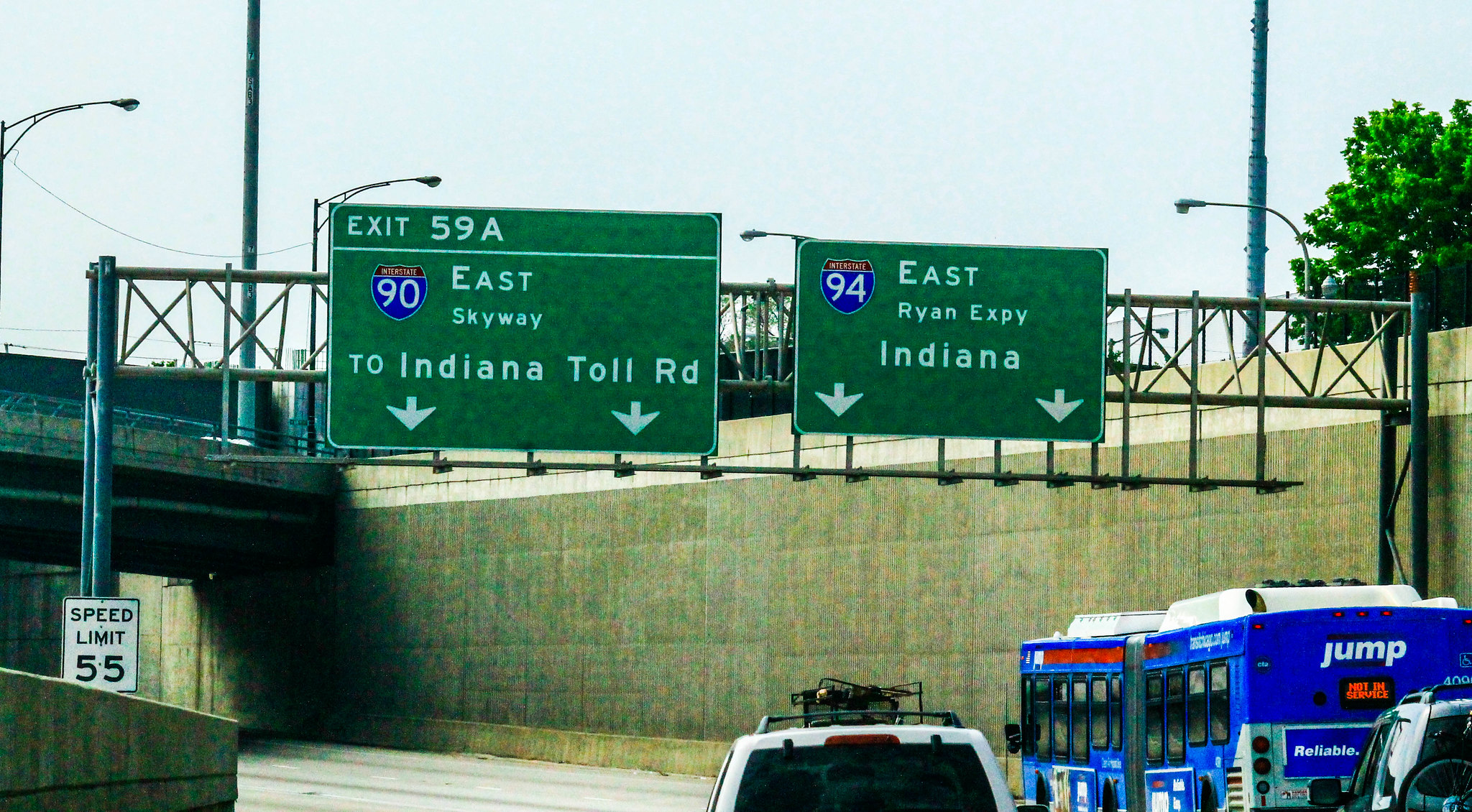This detailed color photograph captures a busy freeway on-ramp scene. Centered prominently is a blue and white articulated bus displaying the words "jump" and "reliable" on its rear, situated in the right lane. Trailing the bus is a black SUV, while to the left lane, a white SUV with a roof rack carrying items is visible. Overhead, green interstate signs mounted on a metal frame direct traffic with clear indications; the left sign reads "Exit 59A Interstate 90 East Skyway to Indiana Toll Road" and the right sign states "Interstate 94 East Ryan Expressway Indiana." A speed limit sign marked "55 mph" is fixed on the lower left. The backdrop features a large concrete wall and a bridge on the left, complemented by a scattered tree on the upper right and utility poles and streetlights stretched across the scene. The sky above is a crisp blue, contrasting with the orderly yet bustling roadway below.